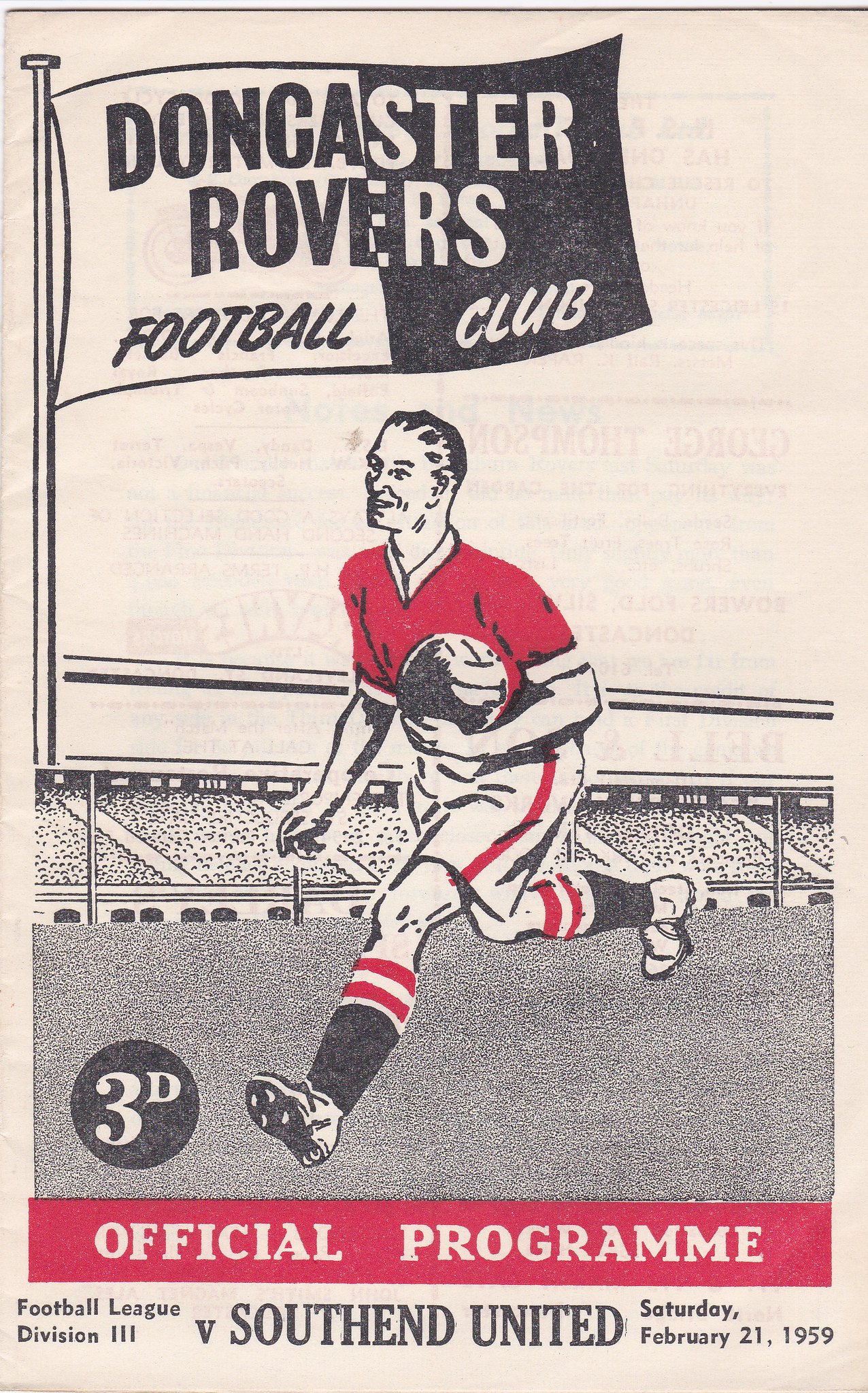This image showcases a vintage illustrated program cover for a Doncaster Rovers Football Club match. Central to the illustration is a middle-aged man, approximately in his 40s, depicted running with a soccer ball. He is clad in a red shirt paired with white pants featuring a red stripe, red and white striped socks, and white shoes. In the upper left corner, a prominent black and white flag bearing the text "Doncaster Rovers Football Club" flutters. The background hints at a soccer stadium filled with an indistinct audience. Below the main illustration, a red banner states "Official Program." Directly above the banner, a circular emblem reads "3D" (likely indicating the price), followed by "Football League Division 3 versus South End United, Saturday, February 21st, 1959" at the bottom. The overall design captures the spirit of 1950s football culture through its detailed and dynamic illustration.